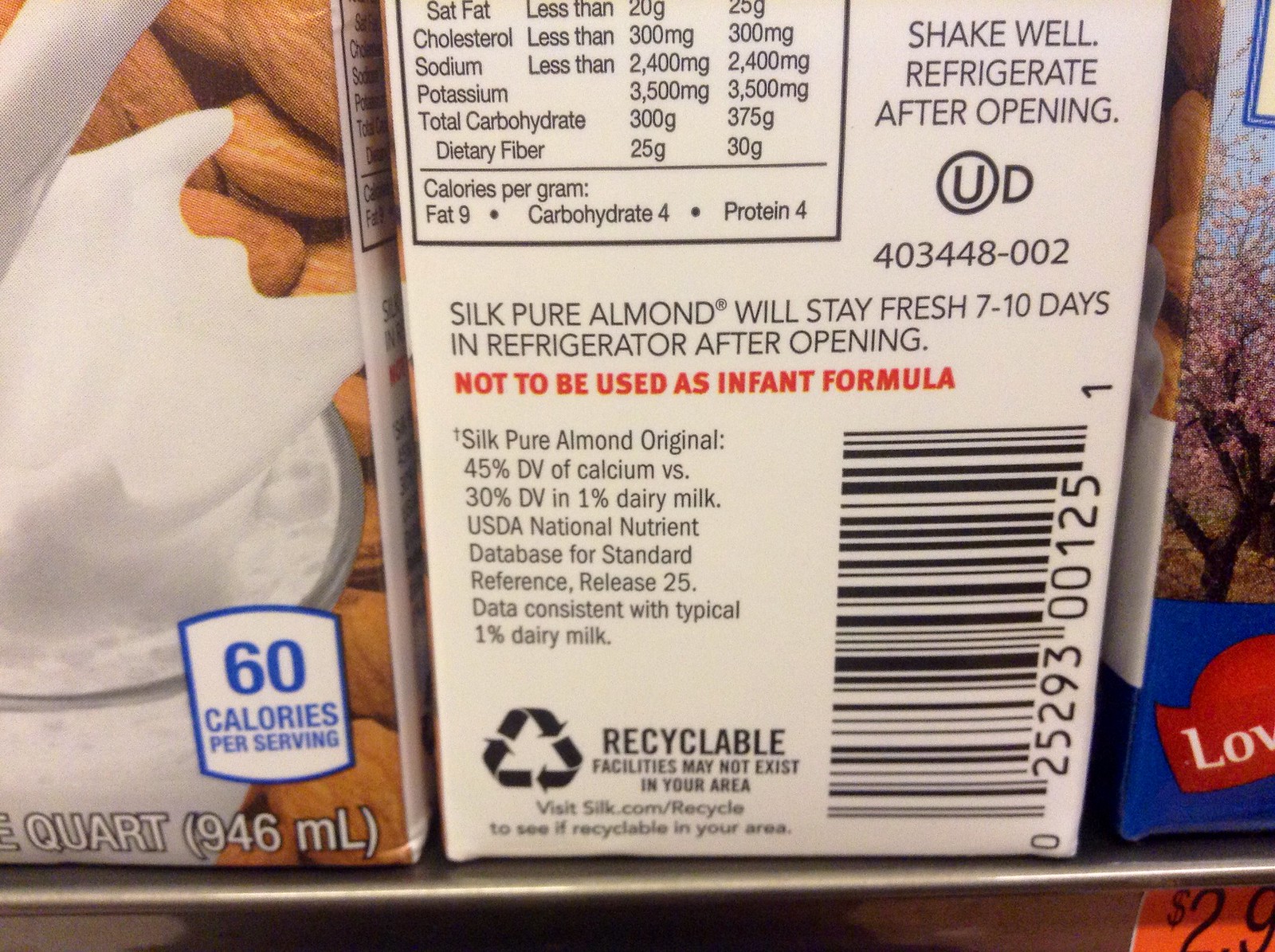This image depicts a close-up view of the back of an almond milk carton on a store shelf, with additional visible packages of almond milk around it. The carton features a detailed nutritional label with specified contents such as saturated fat, cholesterol, sodium, and potassium. Prominent instructions include "shake well" and "refrigerate after opening," along with a note in bold red letters stating "not to be used as infant formula" and that the product "will stay fresh 7-10 days in the refrigerator after opening." The label includes the Silk Pure Almond logo, a circle containing the letter 'U' next to a capital 'D', and product code 403-448-002. 

There is also a notable cross symbol indicating that Silk Pure Almond Original provides "45% D.V. of Calcium versus 30% D.V. in 1% Dairy Milk," according to the USDA National Nutrient Database for Standard Reference Release 25, ensuring data consistency with typical 1% Dairy Milk. The recyclable symbol is present with a reminder to check silk.com/recycle for local recyclability. Adjacent to the barcode number 2529300125, part of an orange price sticker can be seen, stating "$2.9" but cut off at the edge.

Additionally, you can see parts of the packaging featuring images of almonds and a glass of milk with splashes, and a square with a blue border that highlights "60 calories per serving, quart 946 milliliters." The package's front and side elements are visible on the left and right of the image, with text and symbols partially obscured, including a red symbol containing the letters "L-O-V." The scene includes an inch-high glimpse of the top of a silver store shelf, and the surroundings suggest a retail layout.